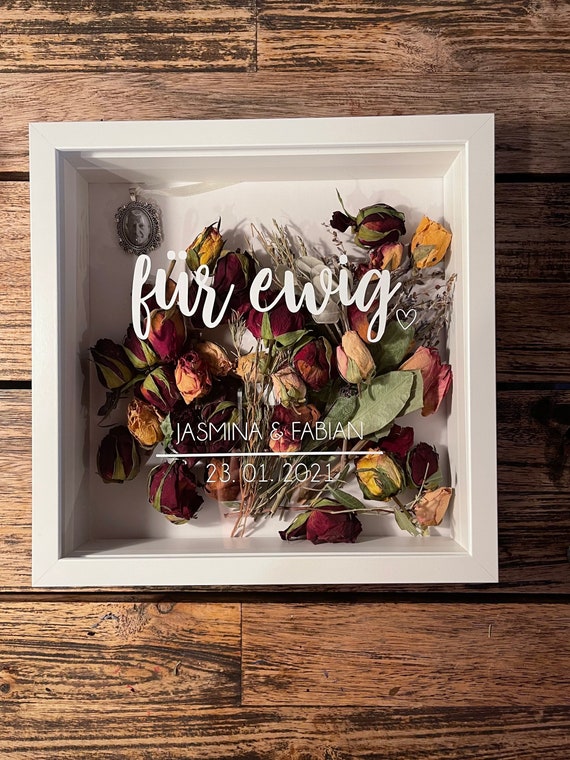The image depicts a white shadow box sitting on a brown wooden surface with visible slats. Inside the box is a collection of dried roses and green leaves, arranged in a way that some are tied together and others are loose. The roses are of various colors—red, yellow, and pink. In the upper left-hand corner of the box is a round, silver brooch, possibly pewter, with a photo of an older man, resembling a locket. The glass front of the shadow box is inscribed with "Fur Ewig" (Forever), followed by "Jasmina and Fabian" and the date "23.01.2021," suggesting it commemorates a significant event. The shadow box appears to be hanging on a wooden wall with horizontal lines between the connecting wood pieces.